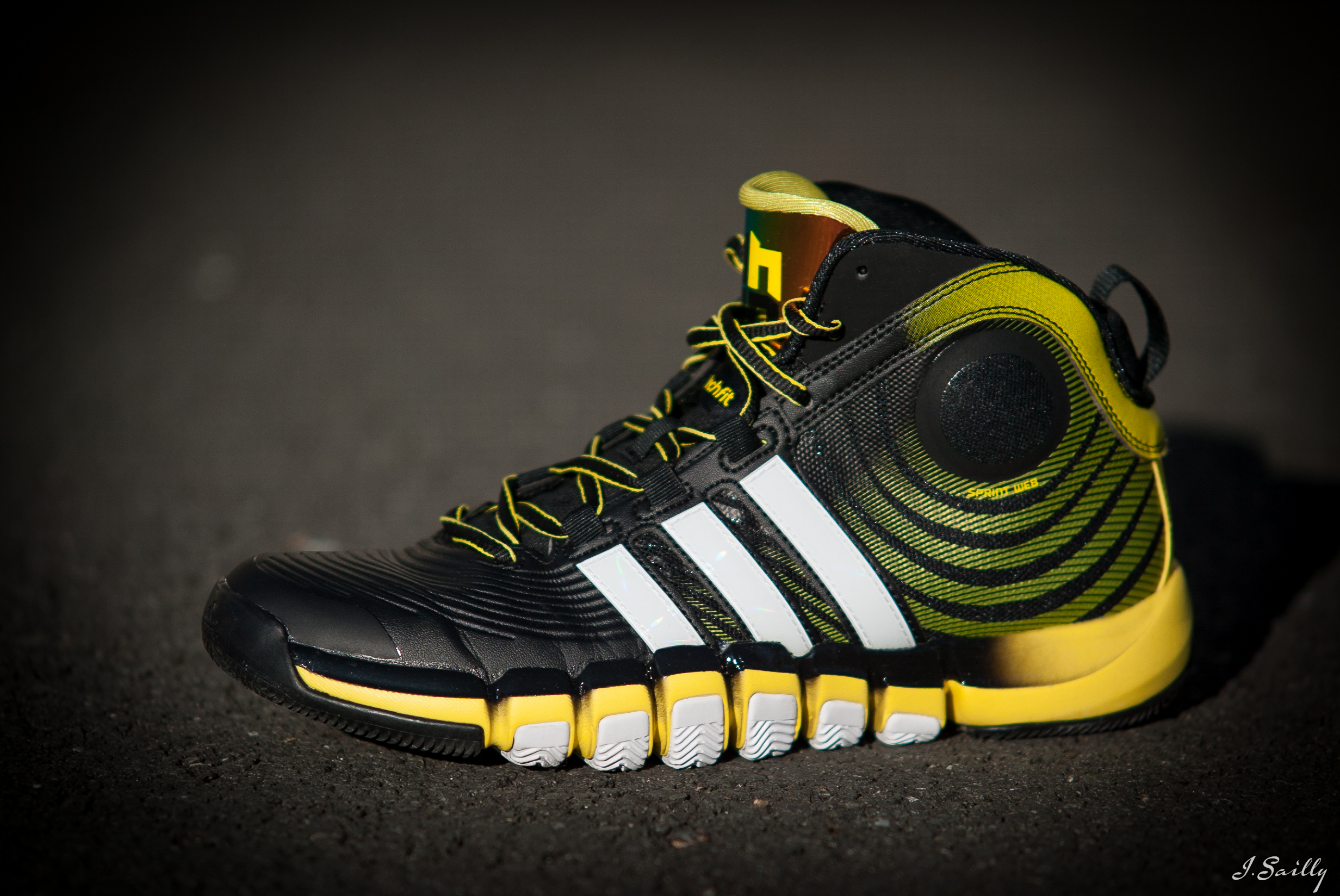This image features a high-top athletic shoe, primarily black, with striking details. The shoe, likely from Adidas given the three white stripes near the black and white laces, has distinct yellow accents. The black tongue of the shoe is trimmed at the top with yellow and features a large yellow lowercase letter, possibly an "H" or "N". The black background emphasizes the shoe, reminiscent of a presentation or advertising setting, with a spotlight on the product. The side view shows a yellow stripe at the front and a wide yellow stripe at the back of the sole, which also has six visible spikes. Bright circular yellow elements and ankle support enhance the rear design. The sole combines black, white, and yellow hues. The overall setup and lighting suggest it's meant for online advertising, perhaps indicated by the text "Jay Salee" at the bottom of the image. The shoe's color scheme and layout give it a bumblebee-like appearance.